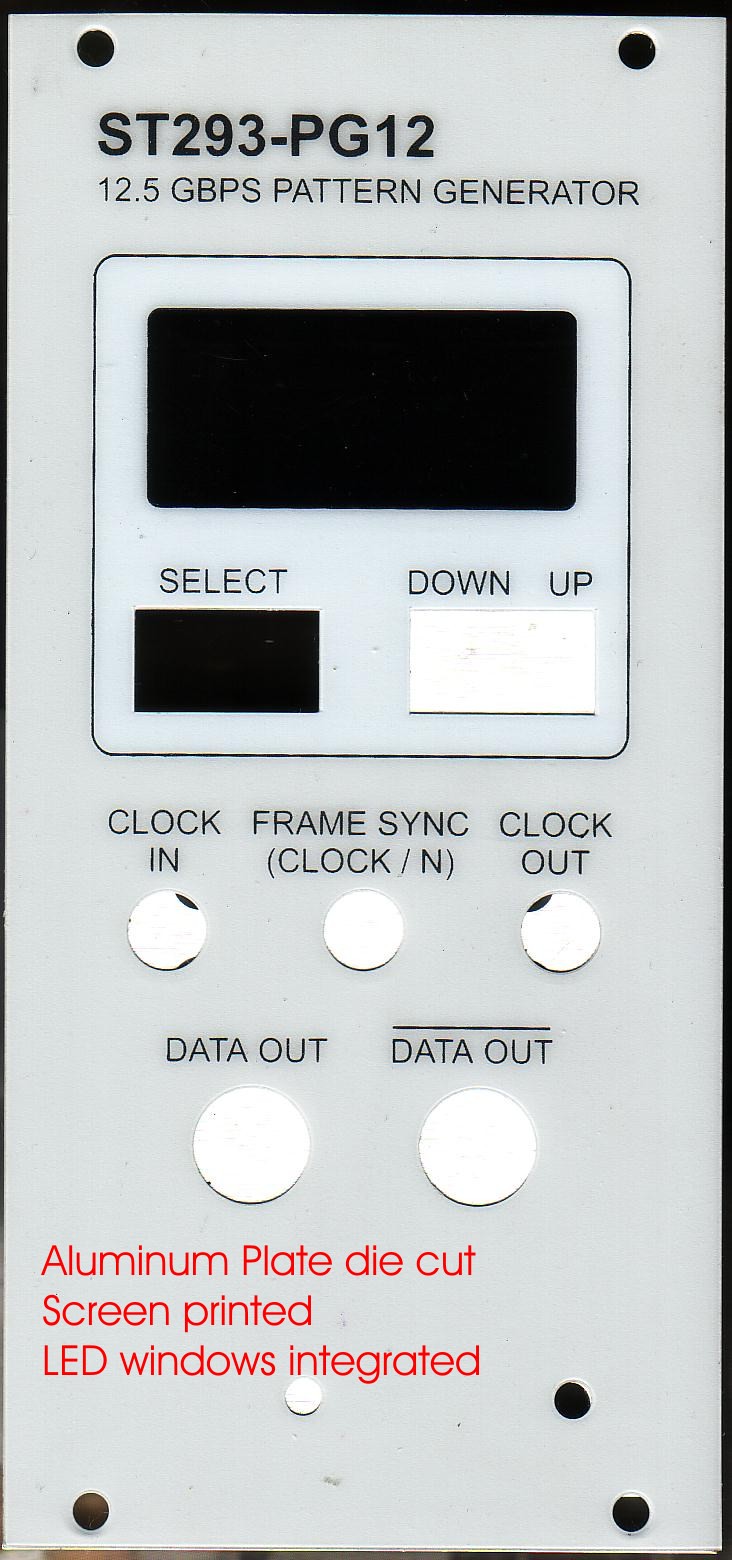The image depicts a sophisticated electronic interface characterized by a sleek, elongated white panel. At the top, the text "ST293-PG12" is prominently displayed in black, followed by "12.5 Gbps Pattern Generator" in smaller font. Below this heading, a bordered black box encloses a white area featuring several labeled sections. 

The first section has a black box with the label "Select" inside it. Directly below, another black box is labeled with "Down" and "Up" controls. Beneath these controls is a white box labeled "Clock In" followed by another white box with the label "Frame Sync Clock In/End." Subsequent to these, there are white boxes labeled "Clock Out" and "Data Out," each indicated with white circular frames. 

An additional white circular frame is positioned above the “Data Out” label. Below the primary elements of the interface, there is red text on an aluminum plate that reads, "Die-Cut Screen Printed LED Windows Integrated." This section is accented by a pattern of small white and black dots arranged in a specific sequence: one white dot followed by three black dots.